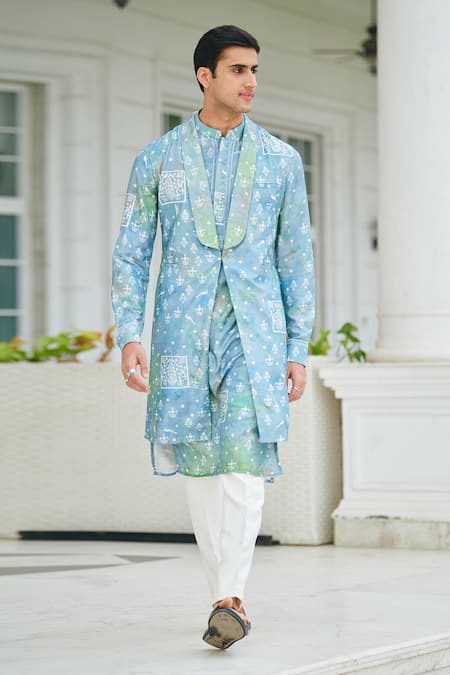A tall, handsome Indian man is captured walking through a courtyard of an opulent white stone building adorned with columns and a large flower box. His slicked-back black hair complements his traditional Indian attire. He wears a beautifully ornate, light blue tunic that extends to his knees, detailed with intricate white and green patterns. Over it, drapes a matching light blue coat. His white slacks peek out from beneath the tunic, ending just above his sandal-clad feet, where his toes are visible. His right hand, adorned with multiple silver rings, swings as he steps forward. The picturesque background, featuring white-trimmed windows and greenery, adds to the impression that this image might be from a fashion shoot. The man gazes off to the left, exuding an air of poise and elegance against the Grecian-style columns and the white marble floor beneath him.